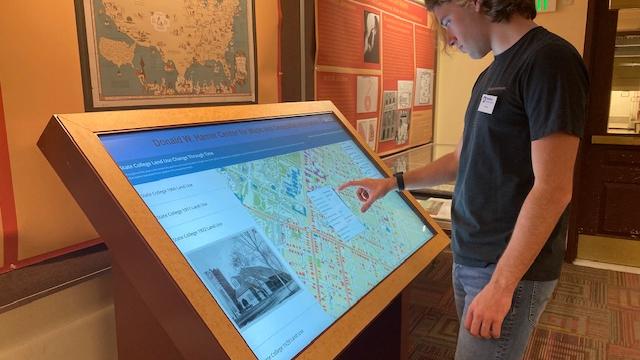In an indoor setting, a young man with shoulder-length hair stands on the right-hand side of the image, wearing a black short-sleeve t-shirt, jeans, and a name tag sticker. He is engaged with a large, interactive touchscreen kiosk, bordered by wood, which displays a lit map and an image of a house or dwelling. The kiosk's screen features a white background with a blue upper layer, and it reads "Donald W. Something Center." Behind him, a framed map of the United States hangs on the wall beside another exhibit featuring a bulletin board area with an orange background, adorned with words and pictures. The area is carpeted, and an exit sign is visible above the man's head. To the right, there is a glass display case with additional items and pictures.